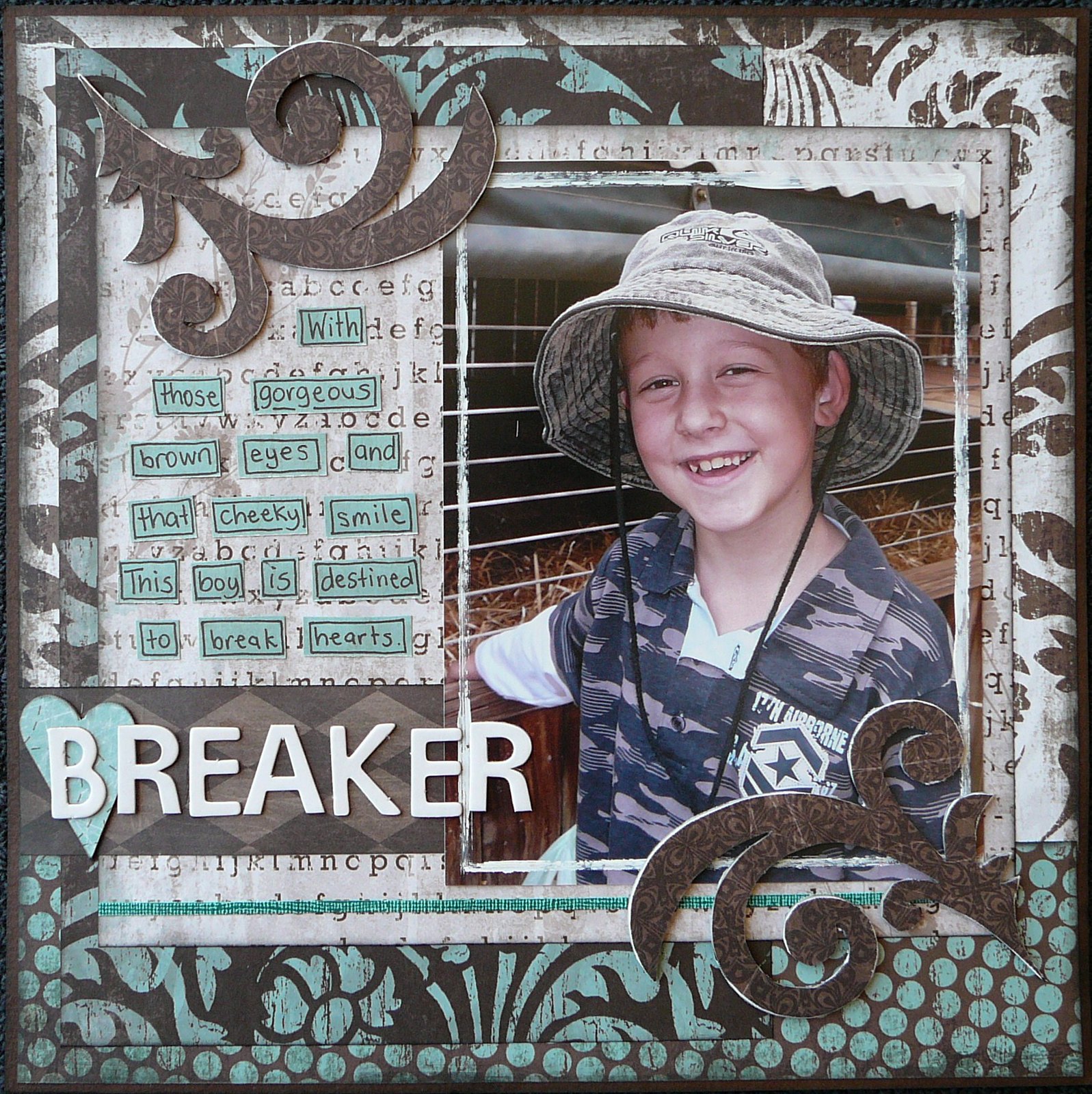This image showcases a square, wooden picture frame with intricate designs and detailed stenciling in light green, teal, brown, and white. The frame holds a rectangular 5 by 7 picture of a young boy, likely between 8 to 10 years old, wearing a fisherman's hat and a long-sleeve shirt with a camouflage design in dark navy and lavender. The picture is positioned to the side, within a background featuring a cream and brown color scheme adorned with floral elements in teal and brown.

The boy, who has his adult teeth in, smiles cheekily at the camera. He possesses gorgeous brown eyes and wears a hat, adding a charming touch to his youthful appearance. Alongside his image, decorative swirling patterns akin to leaves enhance the frame's scrapbook-like aesthetic. To the left of the boy’s picture, in a scrapbook style, the text reads: "With those gorgeous brown eyes and that cheeky smile, this boy is destined to break hearts." Below this sentence, bold white letters spell out "BREAKER," with a light green heart behind the letter "B," further emphasizing the playful and heartwarming captioning. This detailed description comes together to create a picture that is both visually captivating and sentimentally endearing, highlighting the boy's charming personality.